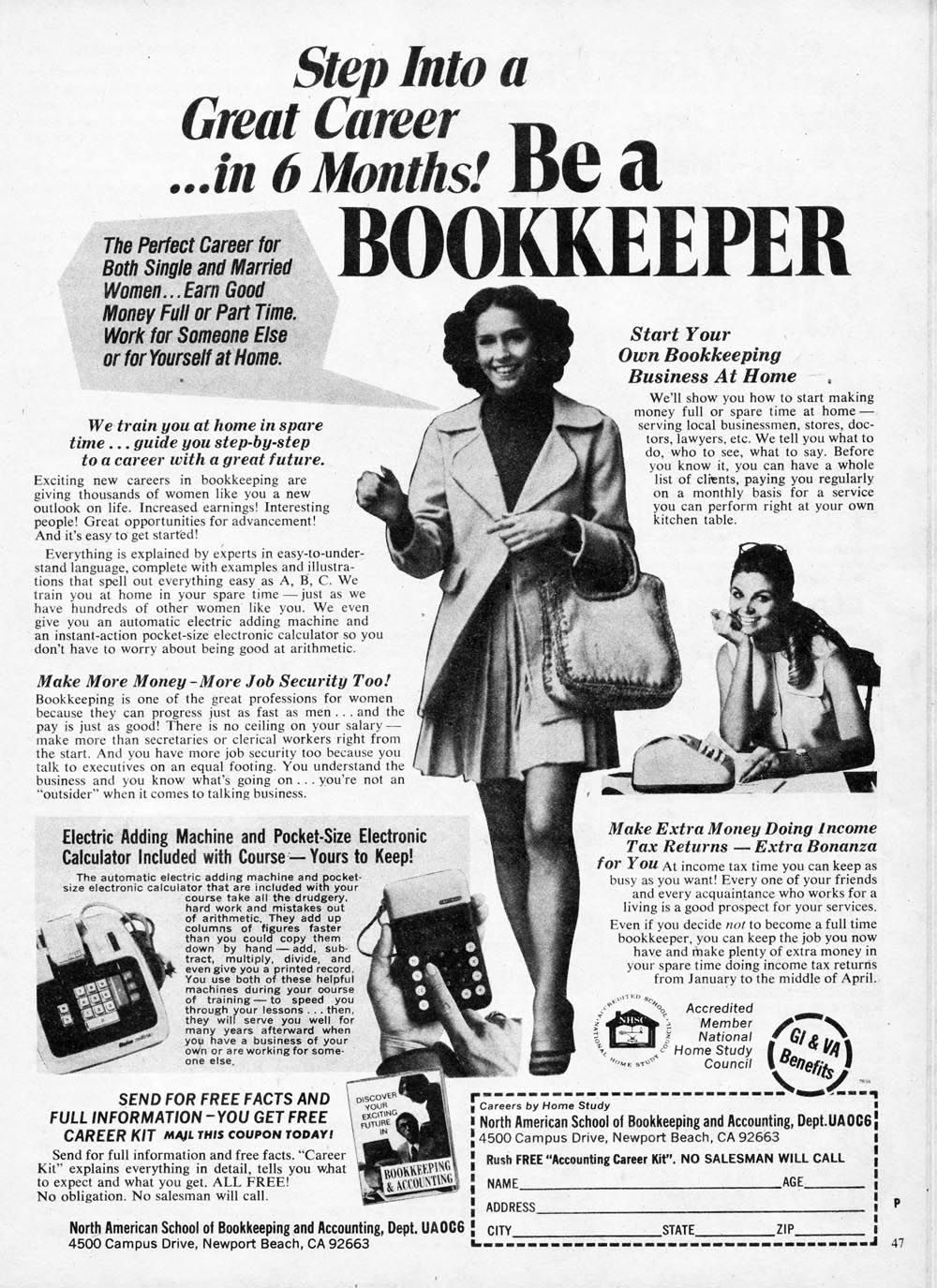This vintage black-and-white magazine advertisement for the North American School of Bookkeeping and Accounting promotes a home study course that promises a career transformation in just six months. The ad’s headline urges, "Step into a great career in six months. Be a bookkeeper." Dominating the center is an image of a smiling woman, stylishly dressed in a jacket and a short skirt that falls above her knees, with heels and a handbag draped over her arm. A speech bubble from her proclaims, "The perfect career for both single and married women. Earn good money, full or part time. Work for someone else or for yourself at home."

The advertisement highlights key benefits of the course, including job security and the potential to start a home-based bookkeeping business. It also encourages making extra money through income tax returns. Enrollments come with an electric adding machine and a pocket-sized electronic calculator for students to keep.

Additional imagery within the ad supports its message, showing a woman at home, happily talking on the phone, alongside smaller illustrations of phones and a book cover titled "Discover Your Exciting Future in Bookkeeping and Accounting." At the bottom-right, a cut-out form offers a "free accounting career kit," emphasizing, “No salesman will call.” The contact details are: North American School of Bookkeeping and Accounting, Department UAO C6, 4,500 Campus Drive, Newport Beach, CA 92663.